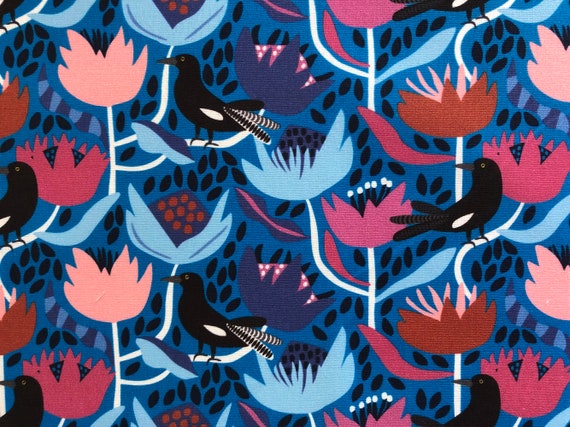In this detailed depiction of a horizontal rectangular image that resembles an artist's drawing or a wallpaper design, a dark blue background showcases a vibrant array of flowers and birds. The vertical white stems support blossoms of various colors - light blue, red, pink, and salmon - arranged orderly across the paper. The flowers feature colorful central parts and are distributed to either side of the stems. Among these blossoms, black birds with varying tail patterns, some all black and others black and white striped, are perched on the stems. The birds appear to be in different states; some seem to be singing. Caterpillar-like shapes are sporadically interspersed among the flowers, adding another layer of detail. Additionally, the background is dotted with small black marks, which could be ornamental, resembling fruits, seeds, or simply an added texture. This artistic piece captures a harmonious blend of flora and fauna, rendered with creativity and intricate detail.